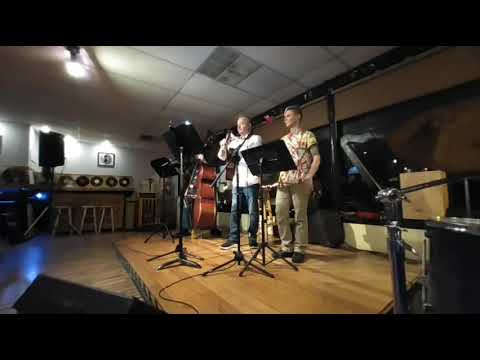The image depicts a group of three musicians performing indoors on a low, wooden stage, situated within what appears to be a bar. The setting is well-lit with both natural light filtering in and a distinct blue light in the distance, complemented by a white ceiling. The stage itself is positioned towards the bottom middle of the photograph and is decorated with black music stands in front of each performer. 

The musician on the right is visible wearing a white shirt paired with blue jeans and appears to be engaging with the audience, although he does not hold an instrument. The central musician is slightly obscured but seems to have a guitar hanging from his neck, actively playing. The third musician, positioned further back, is partially hidden by his large, dark brown bass or cello, which he is in the process of playing.

To the left of the stage, there is a speaker, and visible off-stage elements include vinyl records used as decorations on a bar-like counter with wooden stools. The backdrop includes various indistinct objects adding to the bar ambiance. Overall, the detailed setup suggests a cozy indoor venue with an intimate performance atmosphere.